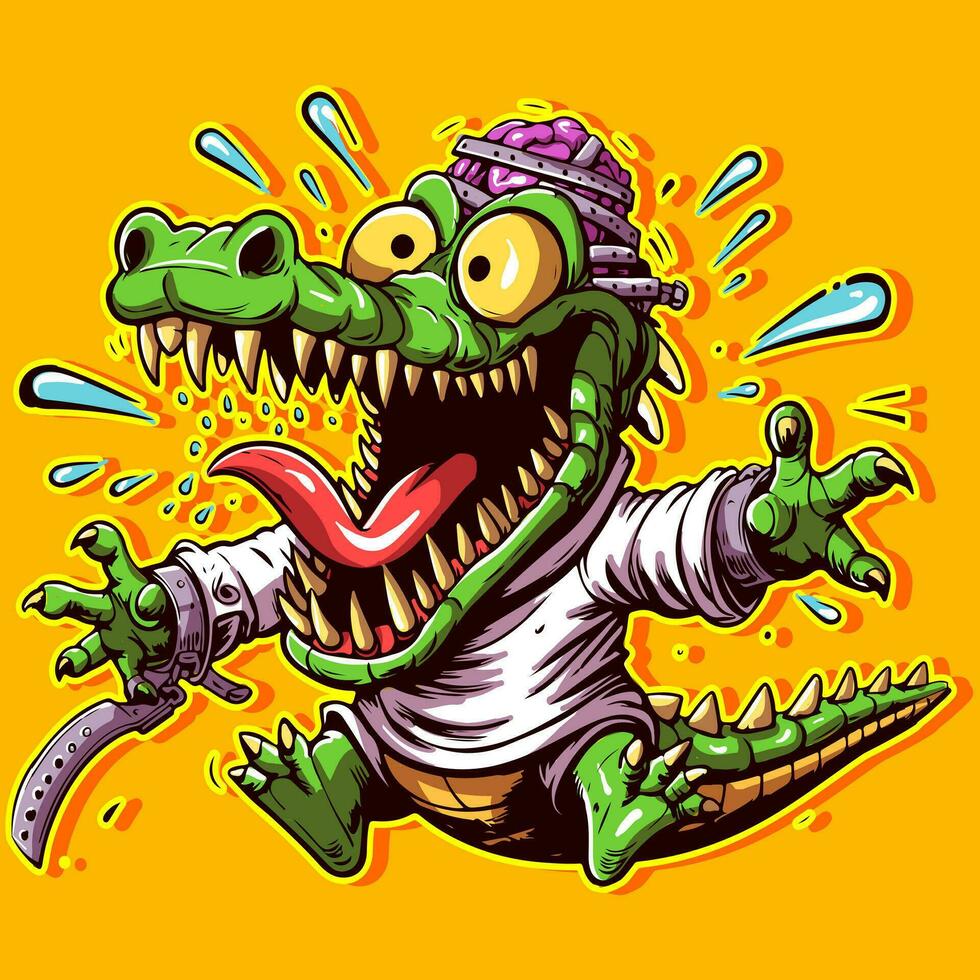This vibrant cartoon artwork features a surreal, giddy, zombie-like alligator character against a bright yellow-orange background. The alligator, or crocodile, sports an excited expression with its mouth open wide, displaying sharp yellow teeth and a red tongue. Bulging yellow eyes convey a sense of exhilaration. Notably, there is an exposed purple brain on top of its head, restrained by metal straps, suggesting a scientific or lab creation. The character wears a white hospital robe, with broken handcuffs around its wrists, implying recent escape from confinement. Sweat droplets and slobber are visibly emanating from its head, enhancing the frenetic energy. Additionally, the creature's arms adorned with clawed hands, a t-shirt with long sleeves, and its tail extending into the background, complete this vivid depiction.